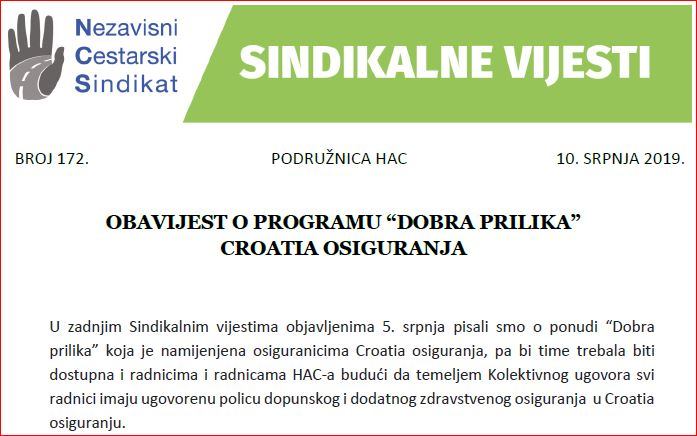The image showcases a predominantly text-based layout, primarily in the Bosnian or Croatian language, suggesting it may be from a website or digital publication. Dominating the center is a block of text, appearing to be an article or newsletter. The headline translates to "Union News," specifying it's from the Independence Sistarskiy Syndicate, issue number 172, dated July 10th, 2019. It elaborates on the Program of Croatian Insurance, mentioning prior coverage in the July 5th edition about an offer dubbed "Good and Opportunity" designed for Croatian Insurance's insured individuals. This insurance policy is available to HAC workers and employees, providing supplementary and additional health insurance as per their collective agreement.

In the top-left corner is a hand holding a picture of a road, creating a unique overlay effect on the text. The color palette includes shades of red, white, blue, gray, light gray, green, black, and multiple instances of white text on the website screenshot. The composite nature of the image, blending a photograph with substantial textual content, suggests it is a digital artifact rather than a conventional photograph, likely captured from a website.